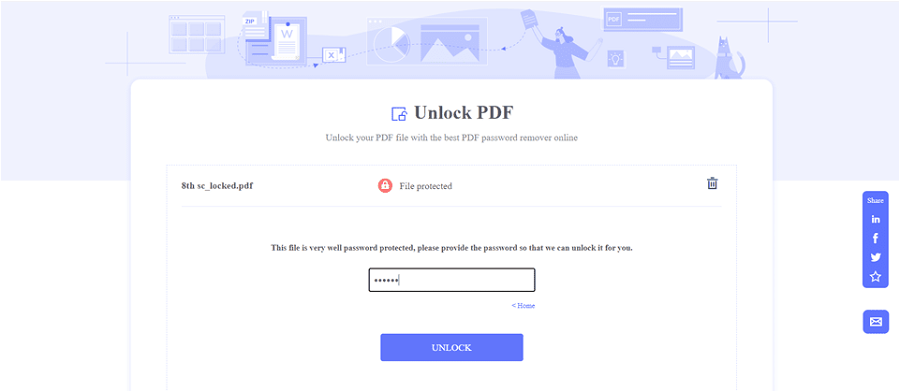Screenshot of an online PDF password remover service. The webpage prominently displays a heading that reads "Unlock PDF" and a subtitle encouraging users to "unlock your PDF file with the best PDF password remover online." An uploaded file named "aethsc.locked.pdf" is shown with a trashcan icon next to it, allowing the user to delete the file if needed. A message below indicates that the file is "very well password protected," prompting the user to provide the password for unlocking. The user is depicted entering the password and is instructed to click the blue "Unlock" button at the bottom. The legitimacy of the service is uncertain, raising concerns about the security of inputting sensitive passwords. In the background, a larger graphic features cartoon drawings of a woman using technology inside a house. To the right, various social media icons for LinkedIn, Facebook, and Twitter are visible, along with an option to bookmark the page.